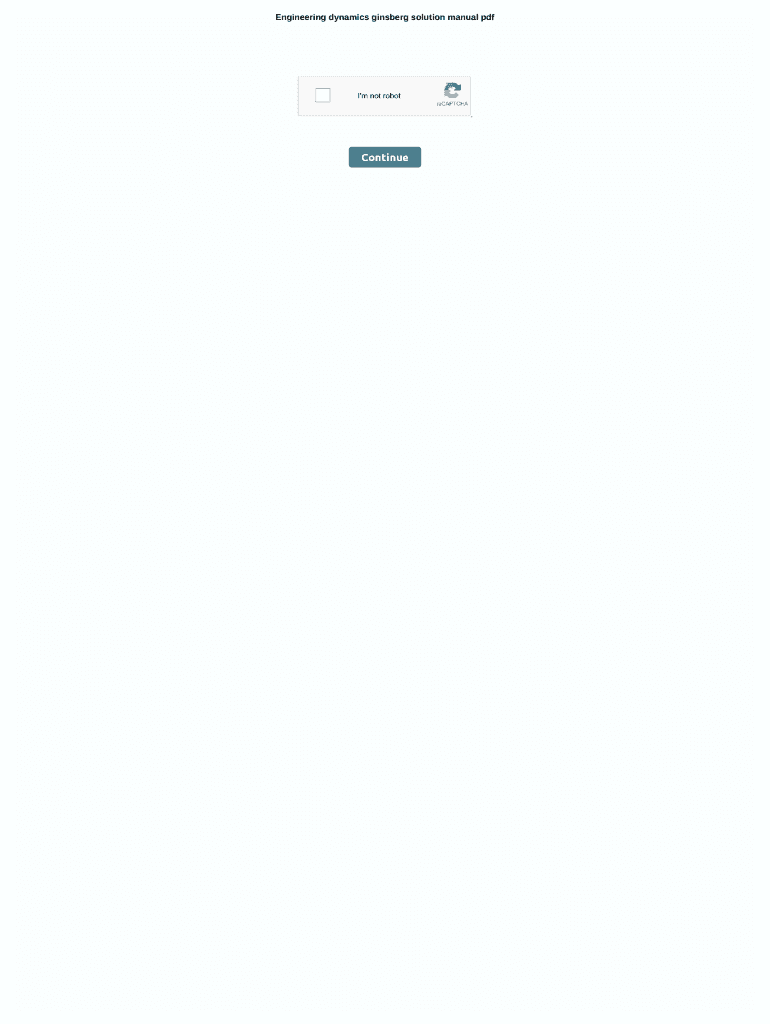**Detailed Caption:**

The image is a screenshot depicting an entire web page with dimensions similar to a standard sheet of paper, approximately 8.5 by 11 inches. The background is completely white. At the very top of the page, in black, bold Arial-type font, is the title "Engineering Dynamics Ginsberg Solution Manual PDF." Below this title is a CAPTCHA verification panel. The CAPTCHA panel is a light gray rectangle contrasting against the white background. Within this panel, there is an unfilled checkbox, which is white. In the center of the CAPTCHA panel, it reads "I'm not a robot" in black text. To the right side of this text is a reCAPTCHA symbol, which features a combination of a curved gray arrow and a curved blue arrow forming a semicircular shape, depicting a rotating motion. Below the CAPTCHA panel, there is a greenish-blue rectangle button with the word "Continue" in white font.